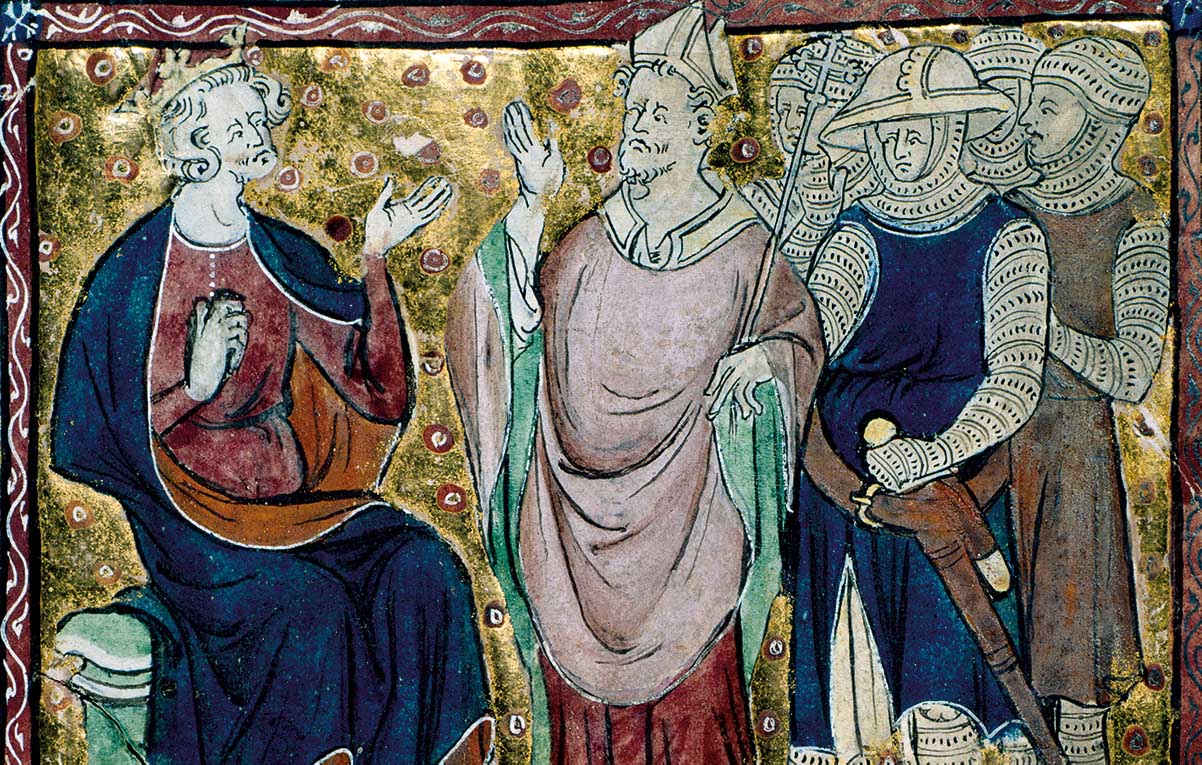The image appears to be a medieval religious illustration showcasing a scene rich in detail and color. At the center, a king sits on a light blue bench, adorned in regal attire with a crown on his head, deep blue robes, and a red shirt underneath. His hand is outstretched in a gesture towards a religious figure standing nearby. This figure is characterized by an ornate triangular hat, a peach-pink robe with green and red layers underneath, and an elaborate collar. He holds a staff and possibly a crown, signifying his importance. To the right, behind the religious figure, stand four military guards, clad in chain mail armor, robes, and helmets, one of whom is visibly holding a sword. The figures are set against a background featuring opulent gold foiling and a palette of rich colors, including deep blues, vibrant reds, browns, and minty greens, encapsulating the medieval art style's richness in a straightforward yet vividly colored scene.